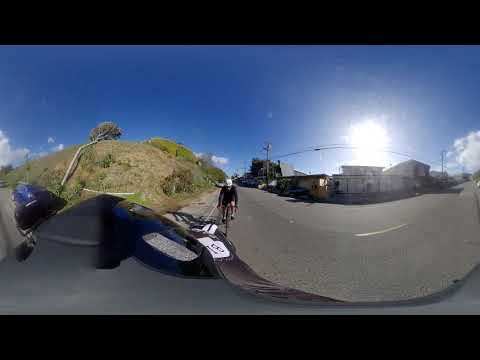This is a digitally altered, cropped photograph taken outside during the daytime, featuring a bicyclist riding down a two-lane road in a residential or semi-rural area. The bicyclist is wearing a white helmet, a long-sleeved black top, and black bike shorts, indicating it’s a warm day. The road has a single white dotted line down the center and there's a grassy, hilly embankment on the left side of the road. The right side features various buildings, possibly industrial, and an altered car either driving down or pulled over to the side of the road. A bright blue sky dominates the image with a single small cloud and a bright white sun partially obscured by power lines. The photograph has black bands at the top and bottom, suggesting it was formatted for digital upload. Additionally, the bottom part of the image shows a secondary overlay with elements like the front of a motorcyclist’s blue helmet and parts of a motorcycle, adding a surreal dimension to the composition.